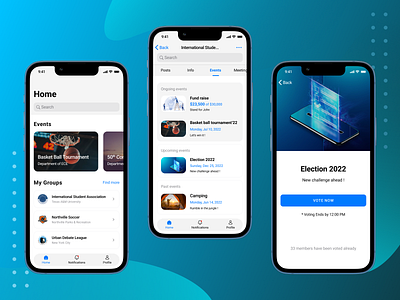The image features a digital depiction of three identical smartphones displayed side by side against a blue background, possibly a computer rendering. The smartphone on the left displays a home screen with options labeled "Home," "Events," and "My Groups," accompanied by screen icons under "Events" and bullet points under "My Groups." The middle smartphone, slightly raised above the others, is grainy and difficult to read but shows four small screen icons with titles beside them, indicating sections such as "Food," "Fundraise," and "Camping." The smartphone on the right showcases an election-themed interface, featuring an image of a ballot going into a slot, with text reading "Election 2022" followed by smaller details about a new challenge and voting instructions. This screen also includes a prominent blue button labeled "Vote now," with a note indicating that voting ends by 12 PM.